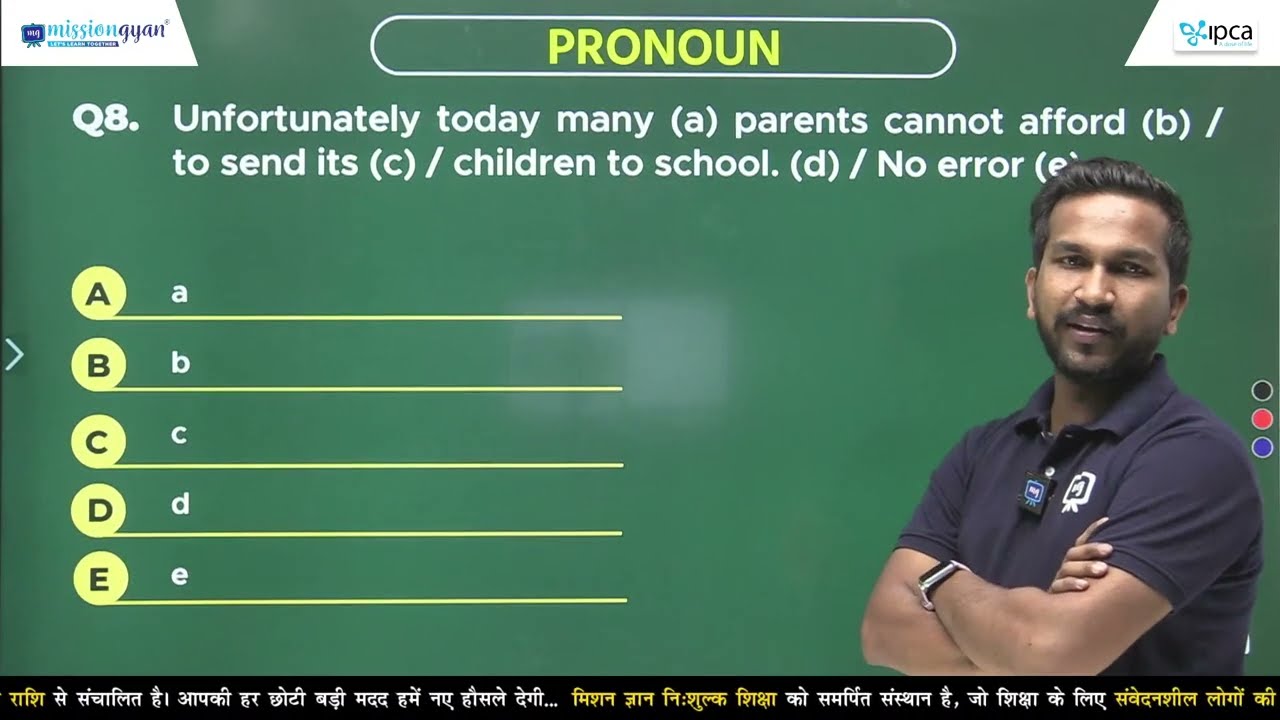In this image, an Indian man with dark brown hair, a mustache, and a beard stands in front of a large green chalkboard. The man, who appears to be an instructor, is wearing a dark navy blue short-sleeved button-up shirt and has his arms crossed, looking directly at the camera. At the top of the chalkboard, within a white rectangular frame with rounded edges, the word "PRONOUN" is written in all capital letters in lime green/yellow. Below it, in white letters, it says "Q8" and features a multiple-choice question: "Unfortunately, today many A. parents cannot afford B. to send its C. children to school D. no error E." The options A, B, C, D, and E correspond to different parts of the sentence, challenging the viewer to identify the correct pronoun usage error. Additionally, there is text in an Indian language at the bottom of the image. The setup suggests an English language lesson focusing on pronouns, likely part of a broader educational initiative, possibly named Mission Gaian.